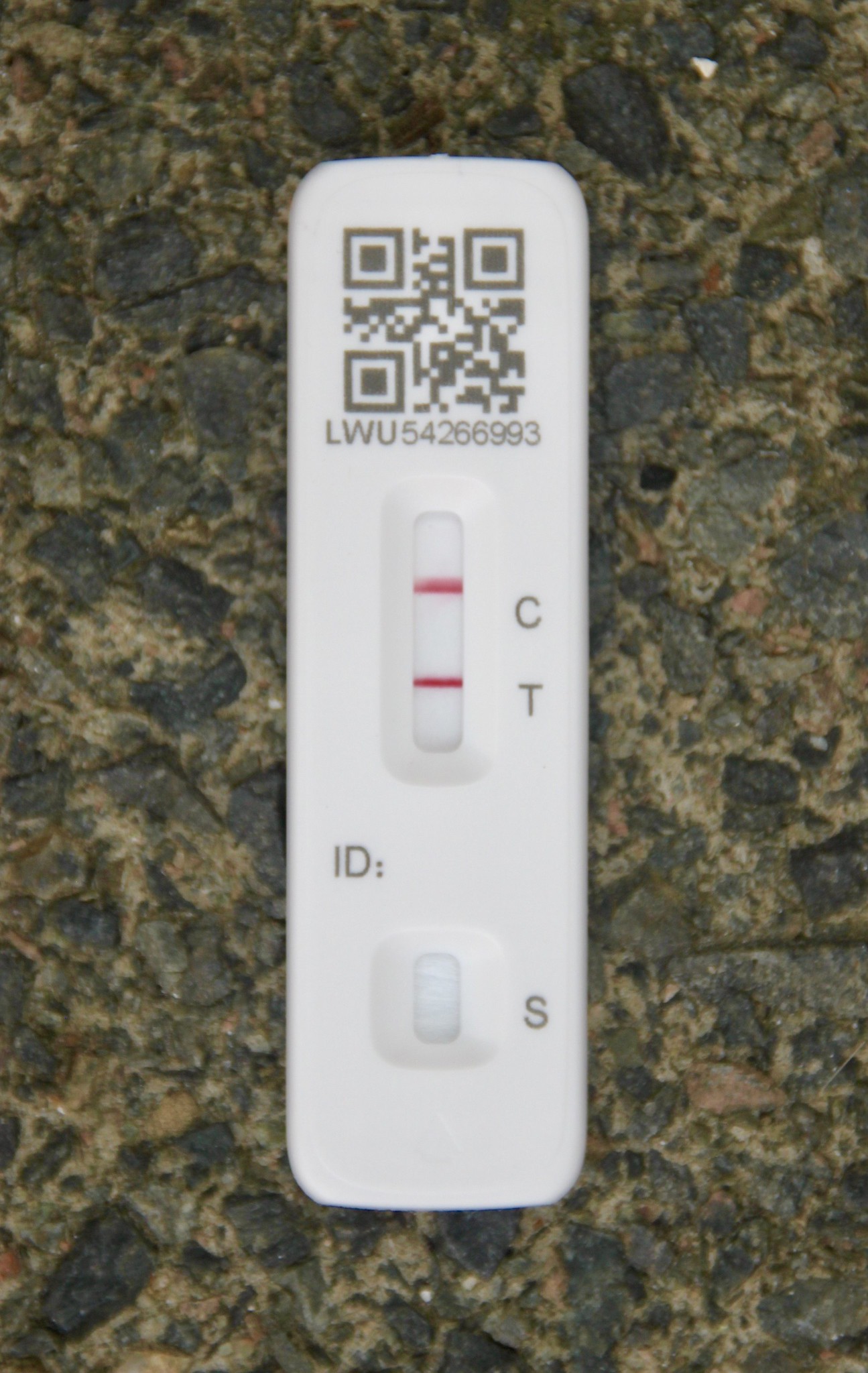A photograph features a positive COVID-19 test resting on a marbled countertop. The counter has a mix of dark gray, tan, light gray, and small flecks of brown. The test itself is a long, white rectangular strip. At the top, there is a black QR code followed by the identifier "LWU54266993" in capital letters. The central portion of the test includes a viewing window marked with "C" above and "T" to the right. Both "C" and "T" have adjacent red lines, indicating a positive result. Below this window, the letters "ID:" are printed next to a smaller empty viewing area, followed by the letter "S" to its right.